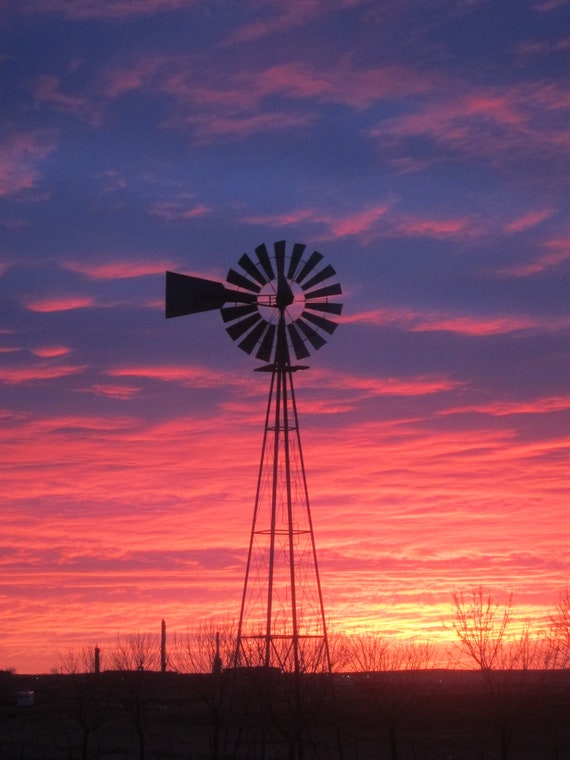This photograph, taken outdoors during either sunrise or sunset, features the striking silhouette of a small farm windmill prominently in the center. The windmill, characterized by a metal frame base and a circular top with many small blades, is fully covered in shadow and faces towards the viewer with its vane sticking out to the left. The foreground includes a row of leafless, barren trees stretching horizontally across the scene, adding texture to the shadowy landscape. The sky above is a breathtaking gradient that transitions from a bright orange and red near the horizon to yellow, and finally to deep purples and blues towards the top, showcasing heavy clouds illuminated by the vibrant colors. In the distance, faint buildings and tiny shrubs can be seen, partially illuminated by the glowing light of the setting or rising sun.